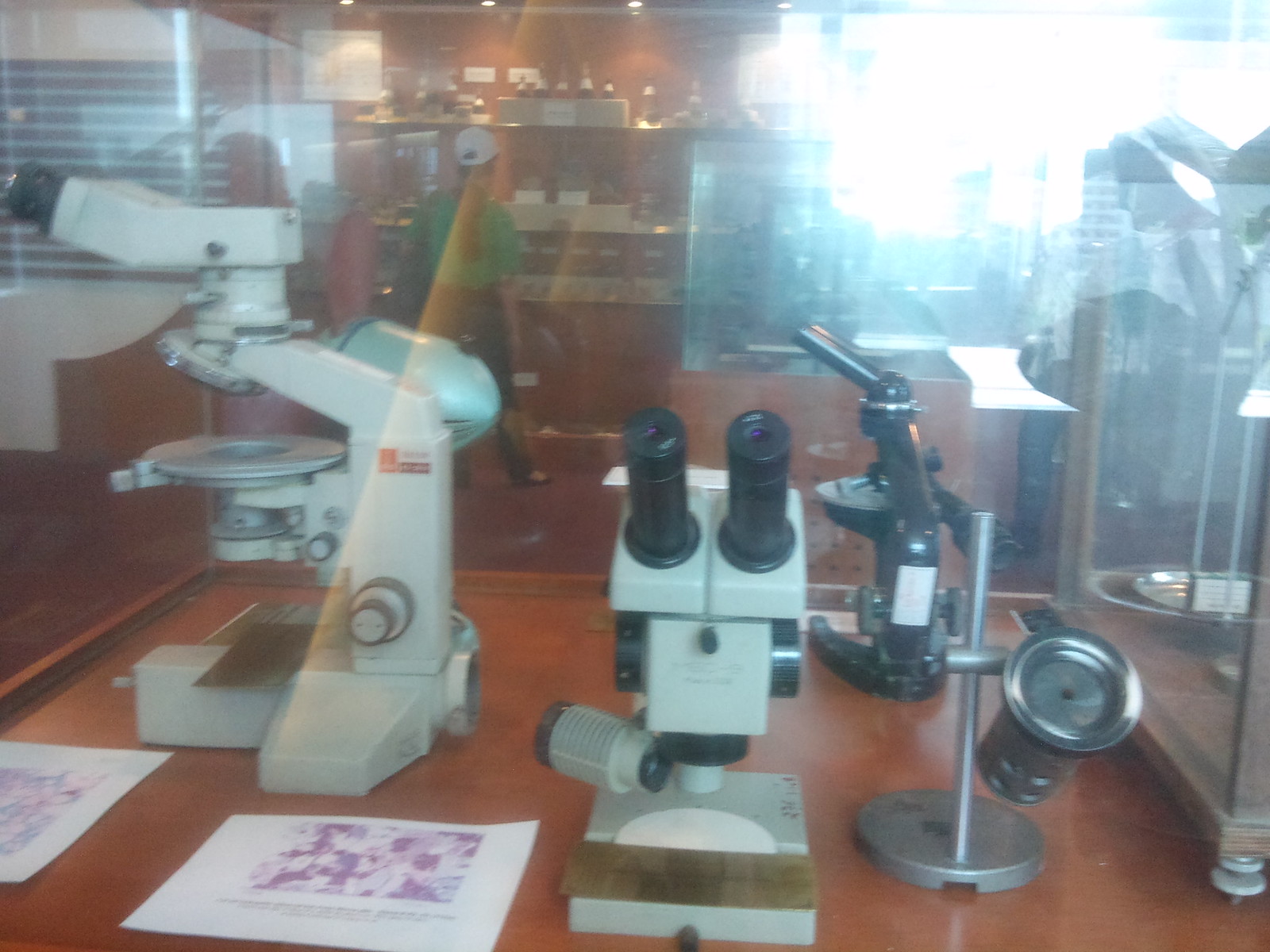The image depicts a well-lit indoor setting that appears to be a lab or a room within a medical or scientific office. Central to the scene are various types of microscopes, ranging from simple models to more sophisticated ones, all positioned on a brown surface. The microscopes are primarily black and white and some are double-lensed. Accompanying the microscopes are several pieces of paper with pictures and drawings, likely used for instructional purposes. 

In the background, partially obscured by the glare of strong sunlight streaming through large glass windows, partitions, and doors, stands a woman. She wears a white baseball hat and a green top, and appears to be looking at items on a shelf. Her lower attire seems to be either black pants or blue jeans, complemented by dress shoes. The sunlight bathes the entire room, creating a bright and almost nostalgic ambiance that suggests the photograph may not be very modern. Additionally, the microscopes and other scientific objects seem to be encased in plexiglass displays, enhancing the sense of an exhibit or a carefully organized workspace. The overall view is slightly distorted, adding to the vintage feel captured by the camera.